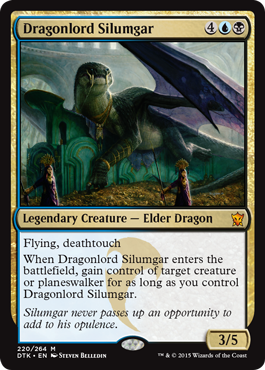This detailed image description is for a gaming card featuring intricate artwork:

The card features a black rim with a gold-based background adorned in black font, prominently displaying the title "Dragonlord Silumgar." Adjacent to the title are three icons: a hammer, a raindrop, and a skull, possibly indicating elements or attributes of the card.

The central image showcases a mythical dragon, Dragonlord Silumgar, in shades of forest green. The dragon, intricately designed, wears a gold necklace and is draped over a large turquoise and gold structure. The dragon's body features a paler green on its neck and belly, with purple wings displaying visible veining. From the dragon's nose area, scaly, string-like elements descend down its body.

Below the dragon, medieval-looking figures, two in number, are depicted. They wear gold and purple robes, wield staffs, and have gold adornments on their heads. The ground in front of the turquoise structure is scattered with gold leaves, adding to the card's opulent aesthetic.

Additional text on the card reads, "Legendary Creature - Elder Dragon," followed by its abilities: “Flying, Deathtouch.” The card explains, "When Dragonlord Silumgar enters the battlefield, gain control of target creature or planeswalker for as long as you control Dragonlord Silumgar." An accompanying flavor text adds, "Silumgar never passes up an opportunity to add to his opulence."

At the bottom of the card, there are numerical values, an artist’s name, a copyright date of 2015, and a numbering indicator of "3/5."